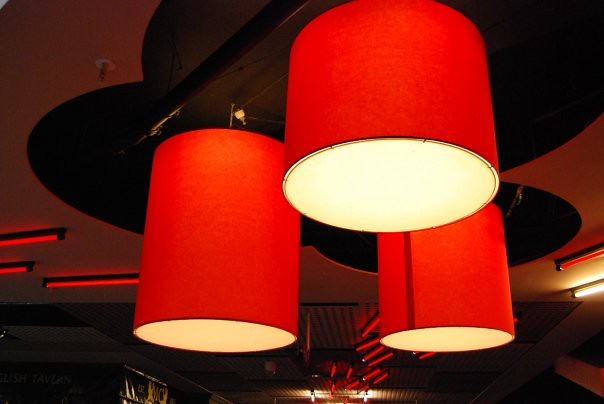The photograph captures an upward-looking view of a dimly lit space, likely a nightclub or bar, featuring an intricate suspended ceiling drop lighting design. Dominating the scene is a large, open section of the ceiling painted dark, shaped like a shamrock or four-leaf clover. From this cutaway, which contrasts with the surrounding red-painted ceiling, three sizable cylindrical lamps hang down, each with a light red, semi-transparent shade. The interiors of these lamps glow with a warm amber or ecru hue, providing indirect, muted lighting. The lamps are suspended from circular black bases, interconnected by visible rods and wires. Scattered throughout the background are additional fluorescent lights, with a mixture of red and white hues, enhancing the ambient atmosphere typical of nightlife environments. The photograph's perspective and the interplay of various light sources contribute to a sophisticated and atmospheric setting.